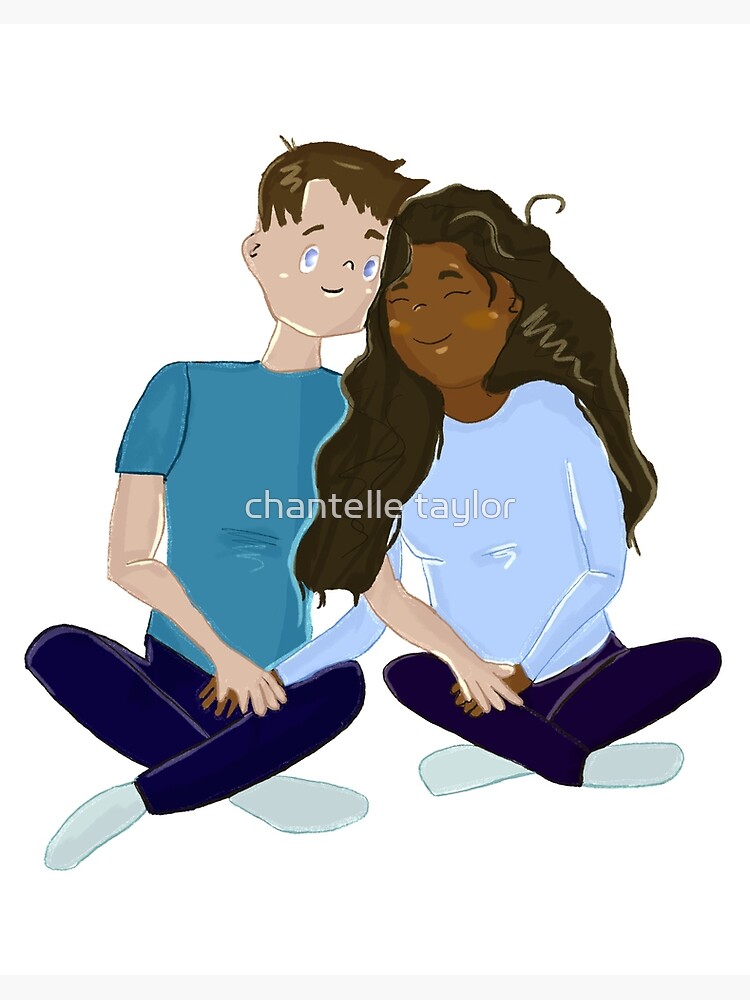This is a digital illustration in a cartoon style featuring a couple of opposite genders and races. Both are seated cross-legged, facing what would be the camera, against a white background. On the left side of the image, there is a white male with short brown hair, brown eyes, and a small nose. He is smiling and has his eyes open. He is wearing a short-sleeve shirt in a shade of blue, purple trousers, and matching socks. On the right, there is a black female with long dark hair, black eyes, and black eyebrows. She is smiling with her eyes closed and resting her head on the man's head. She is dressed in a sky blue long-sleeve top, dark leggings, and sage-colored socks. Their arms are intertwined as they sit close together. The image features a watermark in white that reads "Chantelle Taylor."